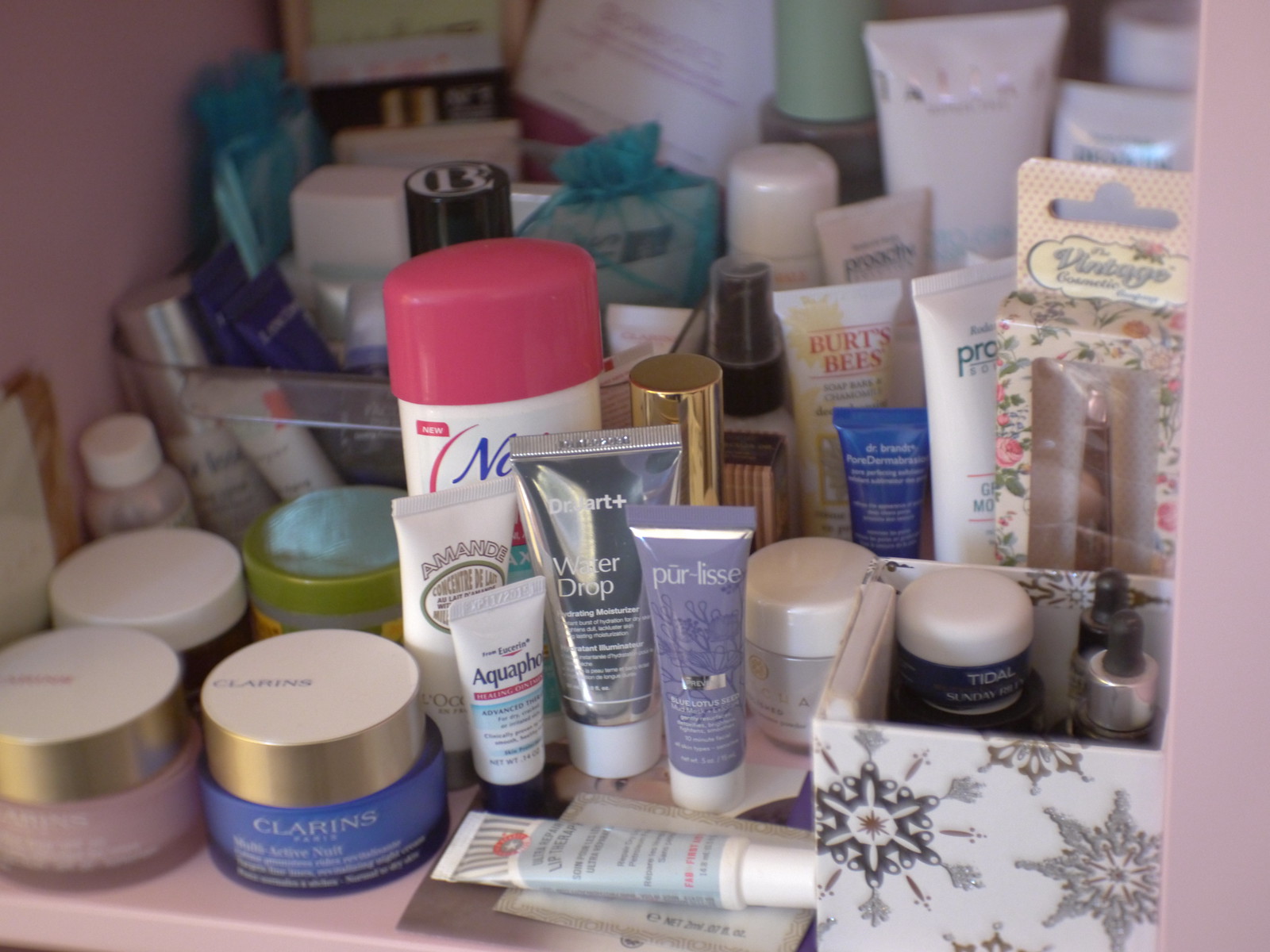In this photograph, an assortment of skin care products is meticulously displayed within a cabinet. The container brims with a variety of items, including many still wrapped in a familiar bag that resembles an Organic Build sample pack. Among the recognizable brands are Proactive Skin Care and Burt's Bees, both in sample and full sizes, convenient enough to carry in a purse. 

The collection also features small containers and vials, such as those for Tidal and Care Lease. Notable mentions include Dr. Art with Water Drop, Aquaphor, and several moisturizers by Clarins. 

These products, which look like drugstore samples, are housed in multicolored jars with prominent product advertising. The array comprises roughly 50 to 60 items, and some remain unopened in their original packaging. In the back, the distinct packaging of Clinique products is also visible, adding to the impressive variety of this skin care collection.